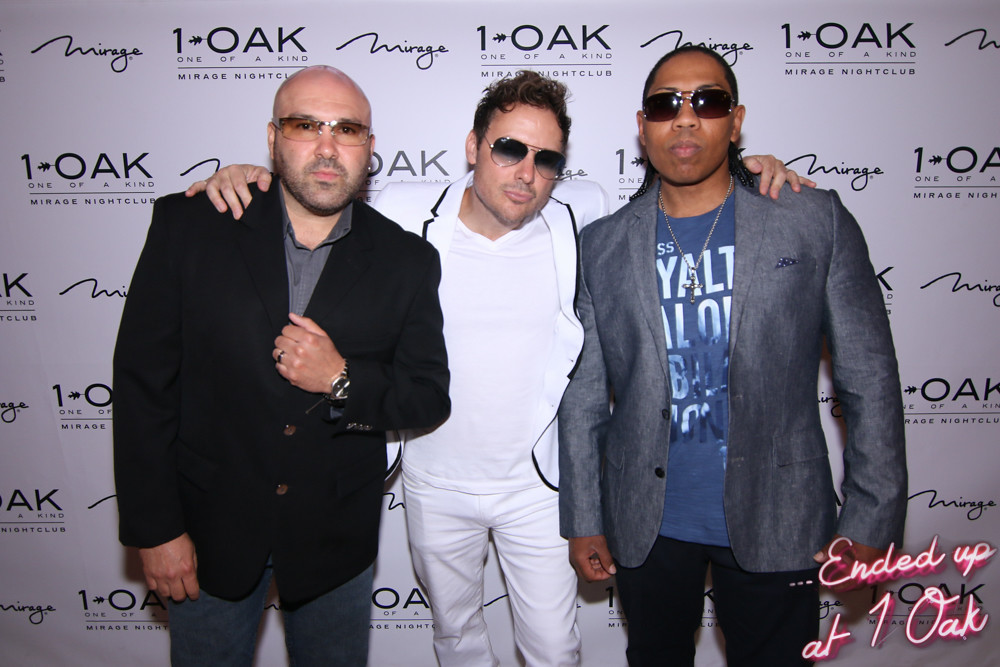In this photograph, three men are standing together with their arms around each other, positioned centrally in front of a repeated logo backdrop featuring sponsorships such as "One Oak" and the "Mirage Nightclub," indicating a promotional or celebratory event, likely held indoors at night. The man on the far left, a white male, is wearing glasses, a gray button-down shirt, dark denim jeans, and a black sports coat. The man in the middle, also a white male, is dressed in an all-white ensemble of a t-shirt, slacks, and a sports coat with black trim, and he sports sunglasses. The man on the far right, an African-American male, is wearing sunglasses, a blue t-shirt with white writing, black pants, and a silverish gray sports coat. The backdrop and their attire suggest a well-dressed appearance suitable for a nightclub or event setting.